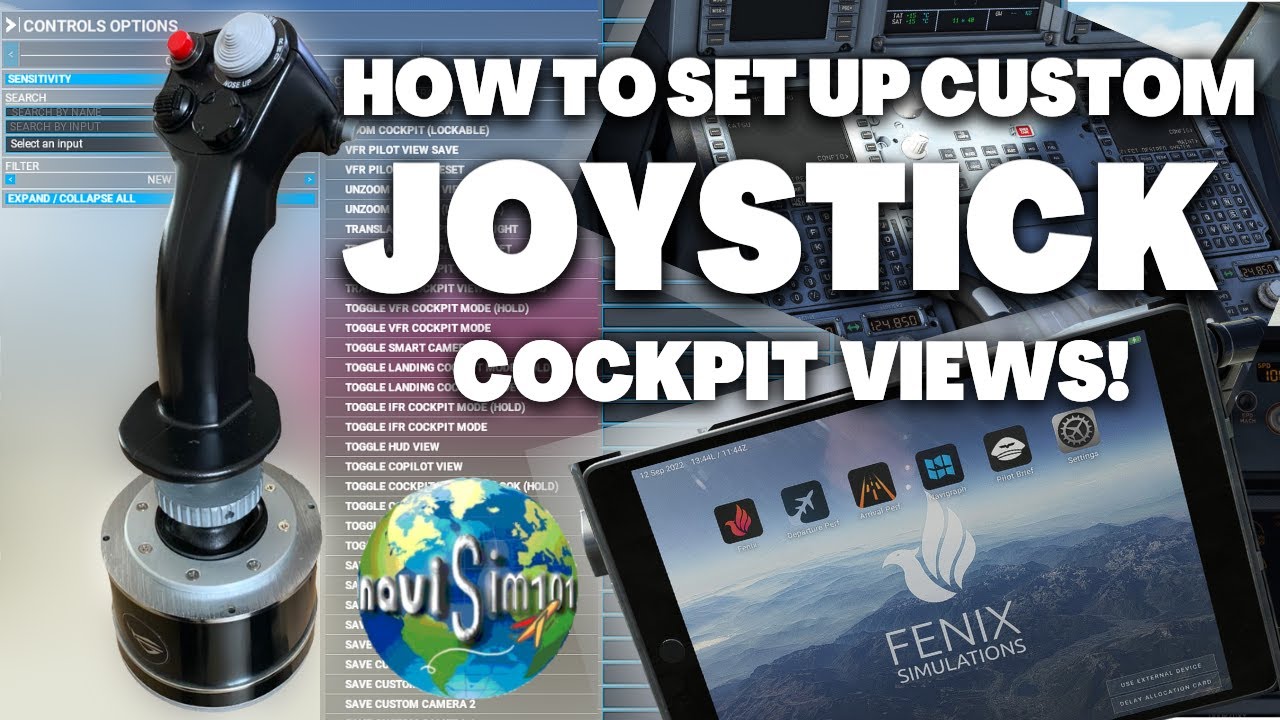In this image, we see a prominent advertisement-like layout that is dominated by large, bold white letters at the top, stating "HOW TO SET UP CUSTOM JOYSTICK COCKPIT VIEWS!" The background is a blend of blue, black, and gray hues, contributing to a high-tech and immersive feel. On the left side, there is a detailed depiction of a black joystick designed for a custom cockpit setup. The joystick features a large gray button, a smaller red button at the top, and is ergonomically curved for hand comfort. Its base is thick and gray with a black rim, and the words "control options" are inscribed in tiny white letters on it.

In the center of the image, there is a blue screen displaying a cockpit background filled with various white textual elements. At the bottom, an earth globe icon, colored in blue and green, is presented with the label "Navi Sim 101." The globe includes the depiction of an airplane route originating from Chile, South America. Additionally, to the right of the globe, there appears to be a tablet-like interface, possibly an iPad, showing several simulated flight applications under the banner "Phoenix Simulations." The overall scene combines elements of aviation simulation technology and detailed imagery to convey information vividly on setting up custom joystick cockpit views.